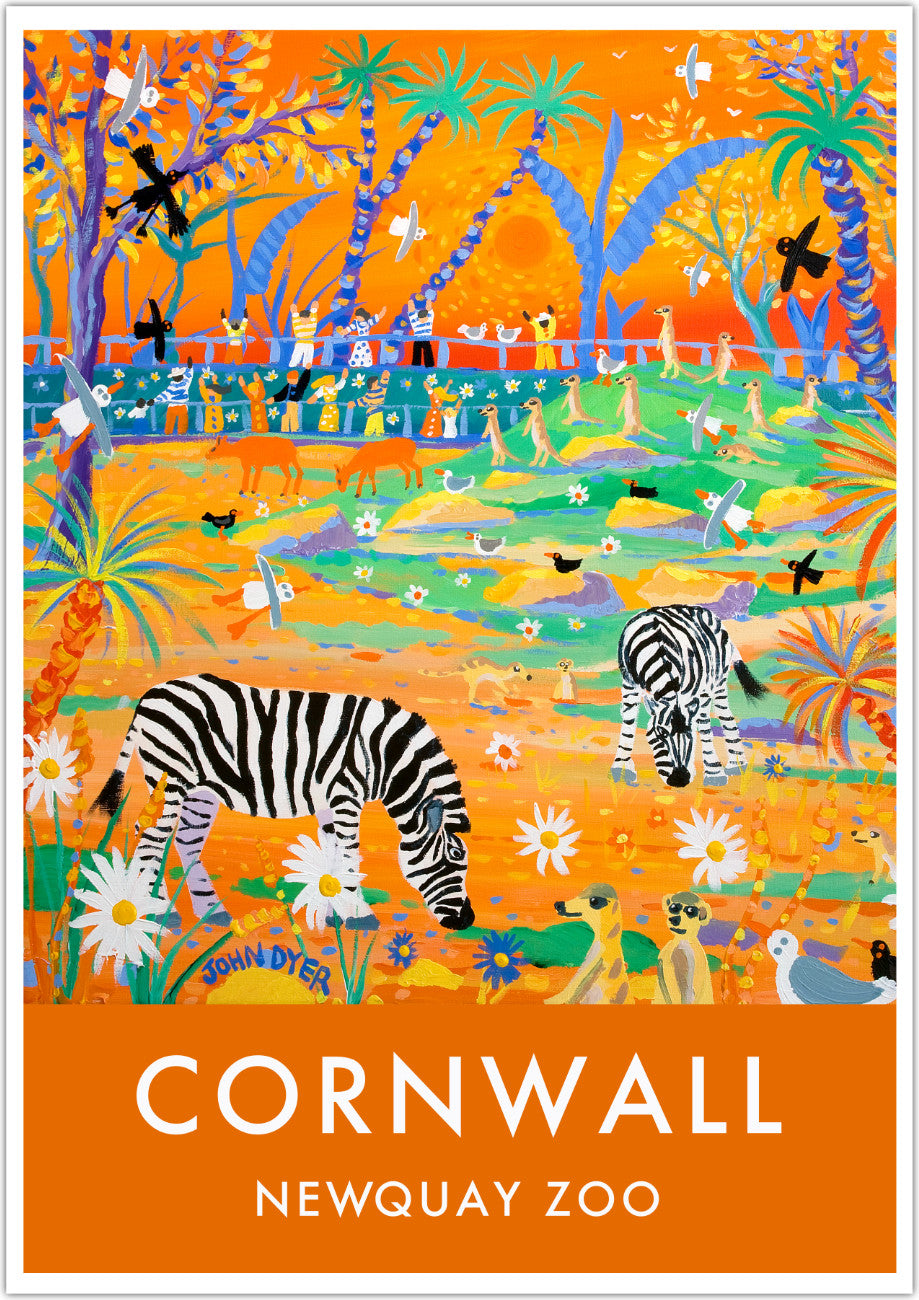This is a vibrant and colorful poster advertising the Cornwall New Quay Zoo. Dominating the bottom quarter of the poster is a solid orange banner, featuring the text "Cornwall New Quay Zoo" in clean, white print. Above the banner, the poster showcases an artistic, comic-style rendering of the zoo's lively environment. The scene includes various animals such as zebras, meerkats, lemurs, ducks, and an assortment of birds in bright, eye-catching colors. Daisies and a diverse array of plants, including creatively colored palm trees with blue trunks and a purple bark tree with blue and yellow leaves, are scattered throughout the image. In the background, behind a blue fence lined with spectators in colorful attire—including yellow and white stripes, floral patterns, and striking dresses—tall palm trees rise against a sky where several birds are depicted flying. The overall composition vividly captures the dynamic and fun atmosphere of the zoo.